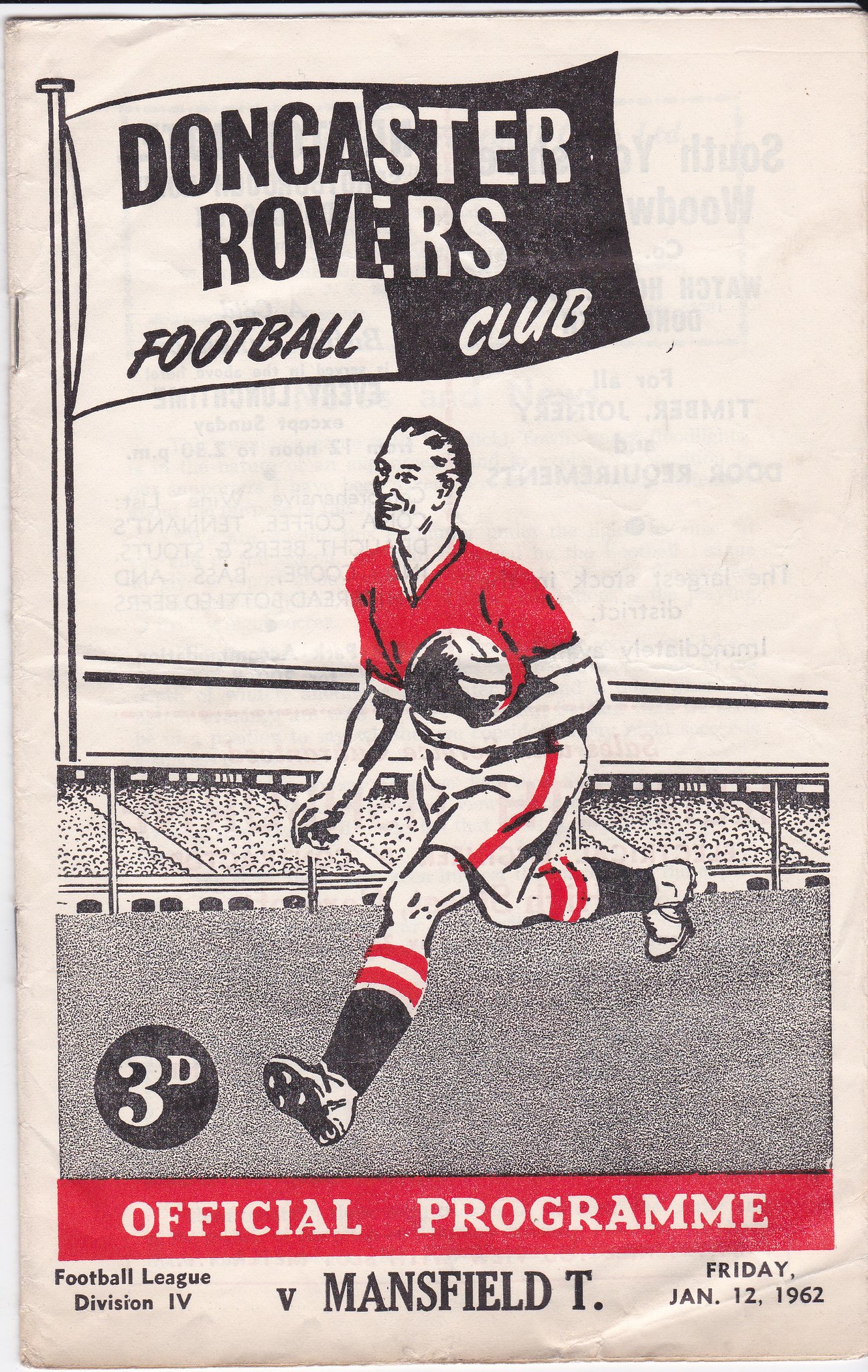This is the front page of an official program for the Doncaster Rovers Football Club dated Friday, January 12, 1962. The cover, weathered and off-white, features an intricate drawing that occupies most of the space. In the upper left corner, there is a flag, half black with white print and half white with black print, bearing the club's name: Doncaster Rovers Football Club.

Dominating the center is the black-and-white drawing of a soccer player in action. The athlete is clad in a red jersey and white shorts with a red stripe along the side. He holds a soccer ball securely in his left hand, preparing to make a play. His legs are in mid-stride, with his right foot forward and his left foot outstretched. The player's knee-high socks are predominantly black, adorned with red and white stripes at the top.

The background is a muted gray, representing the pitch, with stands and spectators faintly visible. At the bottom of the cover, in red text against a white background, it reads "Official Program." Below that, in smaller print, it states "Football League Division 4," followed by "V Mansfield T."